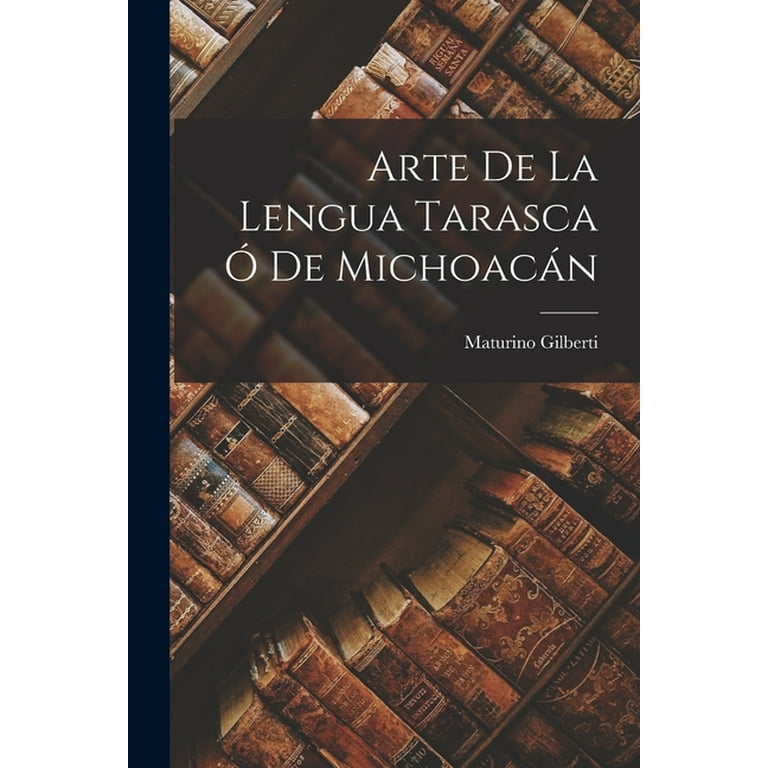The image depicts the cover of a book titled "Arte de la Lengua Tarasca o de Michoacan," authored by Martorino Gilberti. The background features a photograph of a bookshelf filled with ancient, leather-bound books, their yellowed pages and degraded spines arranged at a slight angle. The text on the cover is in white, placed within a gray translucent band across the upper half, with a black band running vertically along the left edge. The color palette includes shades of black, white, rusty orange, and dark red, adding to the antique feel of the cover. The overall design suggests that the book may be about the Tarascan language of Michoacan, although the exact subject is not confirmed.